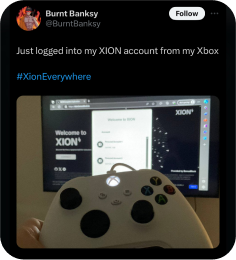The image depicted appears to be a screenshot of a social media post, possibly from Twitter. The visual dimensions of the screenshot form a rounded rectangle that's slightly taller than it is wide. At the top of the image, there's an avatar featuring a cartoon or anime-style illustration of an individual who might be bare-chested or wearing sleeveless attire, standing against a backdrop of flames. The display name associated with this avatar is "Bernt Banksy," and the accompanying Twitter handle is @BerntBanksy. To the right of the username is a white "Follow" button, indicating this is a profile view or an interaction prompt.

Below the header information, the post reads: "Just logged into my Exxon (X-I-O-N) account from my Xbox. #ExxonEverywhere." Accompanying this text is a photograph showcasing an Xbox controller held in front of a screen displaying a website that presumably belongs to Exxon. Although the website text is partially unreadable, the legible portion includes a welcome message: "Welcome to Exxon."